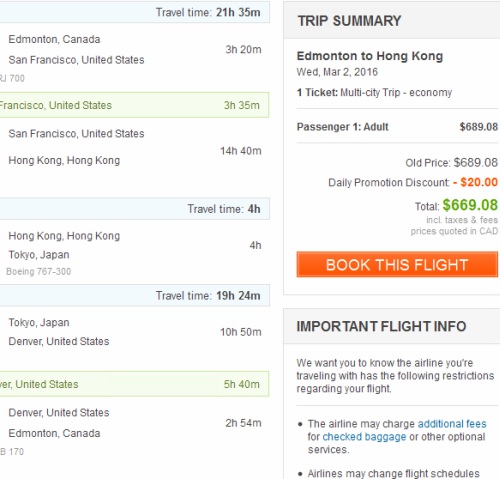This is a detailed caption for an image taken from a travel booking site, showing a complex multi-leg journey itinerary and pricing details:

---

The image displays the results from a travel booking site, highlighting an extensive multi-stop flight itinerary and associated costs. 

**Left Side:**
- **Travel Time:** The total travel time for the journey is noted as 21 hours and 35 minutes.
- **Segments:**
  1. **Edmonton, Canada to San Francisco, United States:** Duration 3 hours and 20 minutes.
  2. **San Francisco, United States:** Layover duration is 3 hours and 35 minutes.
  3. **San Francisco, United States to Hong Kong, Hong Kong:** Duration 14 hours and 40 minutes.
  4. **Travel Time Placeholder Segment:** The notation "Travel time 4H" is highlighted in a light blue bar, referring to a break or transition period.
  5. **Hong Kong, Hong Kong to Tokyo, Japan:** Flight duration of 4 hours on a Boeing 767-300.
  6. **Next Travel Time:** Another period noted as 19 hours and 24 minutes.
  7. **Tokyo, Japan to Denver, United States:** Flight duration of 10 hours and 50 minutes.
  8. **United States Segment:** A break or layover denoted as 5 hours and 40 minutes.
  9. **Denver, United States to Edmonton, Canada:** Duration 2 hours 54 minutes.

**Right Side:**
- **Trip Summary:**
  - **Route:** Edmonton to Hong Kong.
  - **Date:** Wednesday, March 2, 2016.
  - **Booking Details:** One ticket for a multi-seat trip in economy class for one adult.
  - **Pricing:** Initial price - CAD 689.08. Daily promotion discount of CAD 20 is highlighted in red, leading to a new total of CAD 669.08, including taxes and fees. 
  - **Currency:** Prices are quoted in Canadian Dollars (CAD).
  - **Action Button:** The image features an orange rectangle with the text "Book This Trip."

- **Important Flight Info:** The image includes a note about airline restrictions, stating that the airline may charge additional fees for checked baggage or other optional services. It also cautions that flight schedules may change.